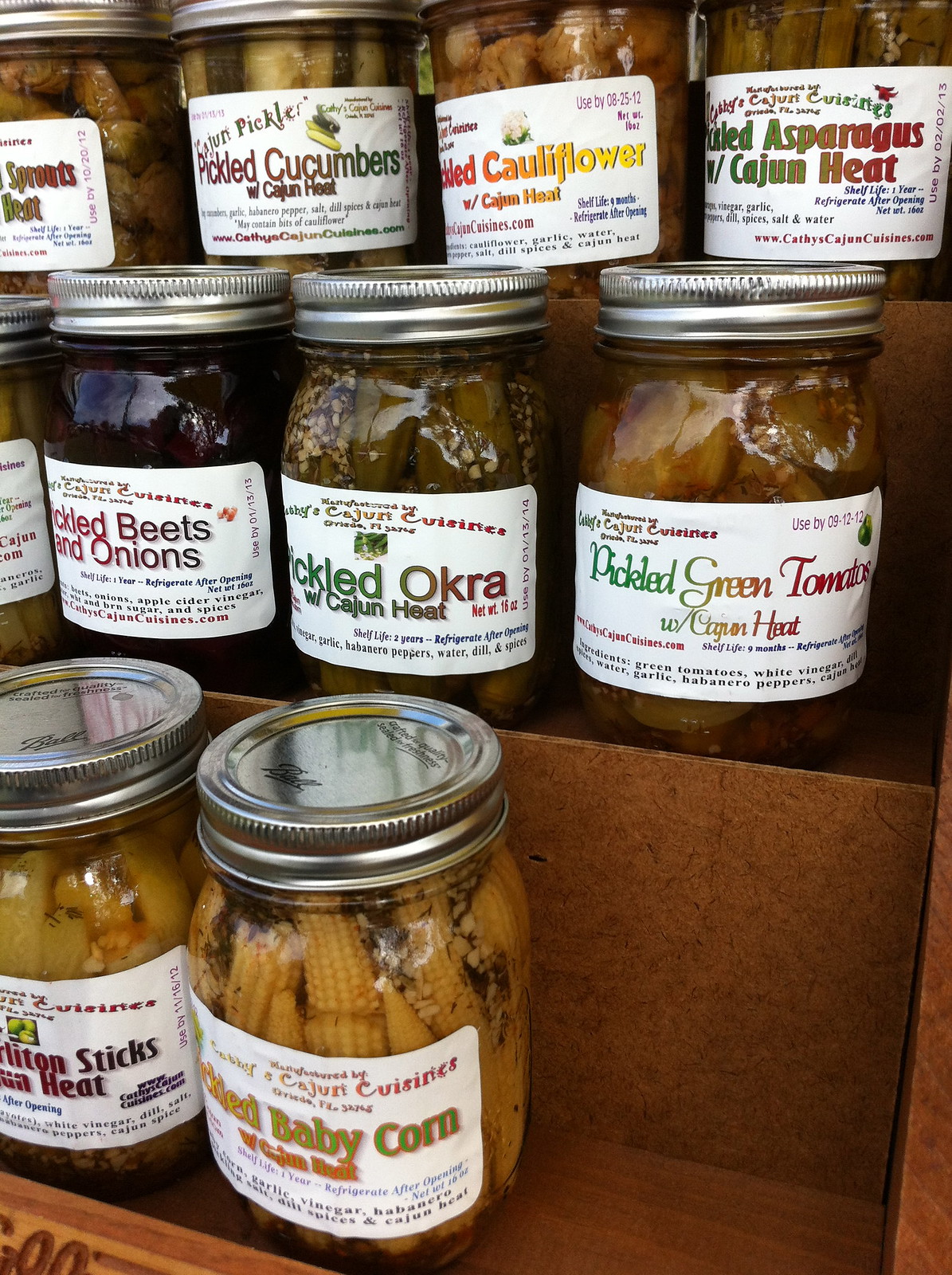The photograph captures an eerie outdoor setting featuring a vertically rectangular, medium-brown wooden shelf with three levels, each filled with an assortment of pickled vegetable jars. The jars, uniform in size, are made of clear glass with silver metal lids and adorned with white labels. Each jar displays the logo "Cathy's Cajun Cuisine" alongside detailed descriptions of their contents and instructions such as "refrigerate after opening."

Arranged from top to bottom and left to right, the top row of jars includes products like pickled cucumbers with Cajun heat, pickled cauliflower with Cajun heat, and pickled asparagus with Cajun heat. The middle row holds jars of pickled beets and onions, pickled okra with Cajun heat (net weight 16 fluid ounces with a three-year shelf life), and pickled green tomatoes with Cajun heat (with a nine-month shelf life). The bottom row features jars labeled pickled baby corn (net weight 16 ounces with a one-year shelf life) and an obscured product likely indicating "sticks with Cajun heat."

The image, reminiscent of a DIY or homemade setup, captures the rustic, handcrafted essence of these pickled goods against the backdrop of the eerily tranquil outdoor setting.